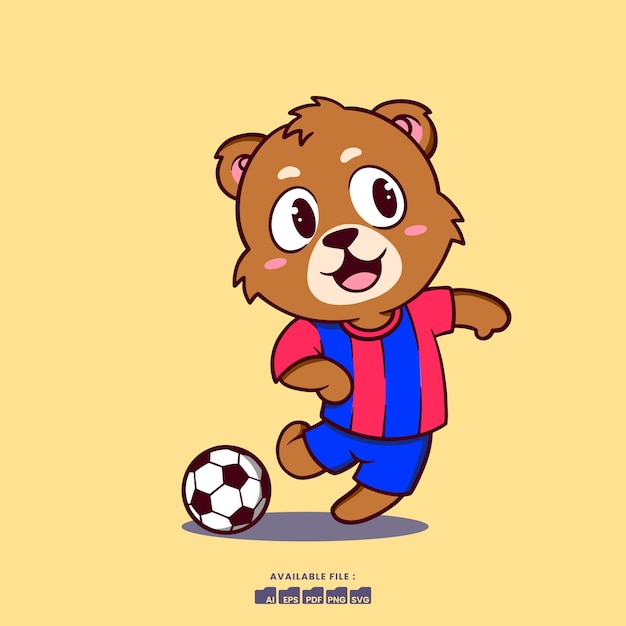Image Description: 

This image is a clip art style cartoon illustration set against a tan square background that features a gradient from darker tan at the top to lighter tan at the bottom. The central character is an anthropomorphic young brown bear with a large head and small body, a common trait in cute cartoons to denote youth. The bear has endearing, big anime-style eyes, pink inner ears, pink blush highlights on its cheeks, a pink tongue, and a circular beige patch around its black nose and mouth. It is smiling warmly. The bear is dressed in a vertically striped red and electric blue soccer jersey, paired with matching electric blue shorts. 

In the scene, the bear is poised to kick a soccer ball, which is depicted to the left of the bear near the bottom of the image. Both the bear and the soccer ball cast round shadows on the ground beneath them, adding a sense of depth. 

Beneath the bear and the soccer ball are watermarked text and icons indicating the availability of the image in several file formats: AI, EPS, PDF, PNG, and SVG.